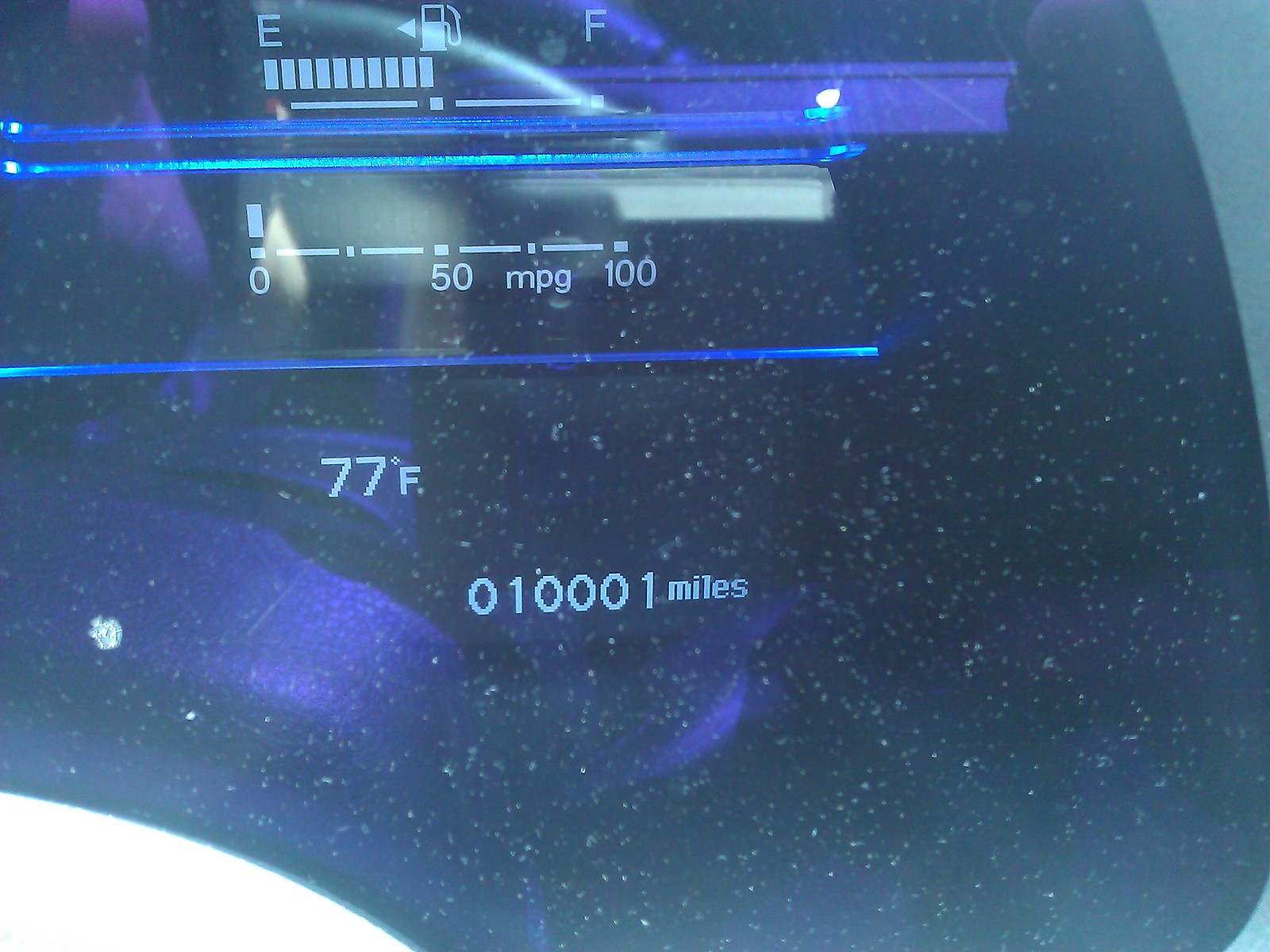The image shows a close-up of a modern car's digital dashboard display, predominantly colored in blues and grays, with a few areas of glare and noticeable dust on the surface. At the very top of the screen, there's a gas gauge with a gas pump icon indicating the tank is half full, located between the "E" (Empty) and "F" (Full) markings. Below the gas gauge, there’s a metric labeled "MPG" and "0-100," suggesting it has to do with miles per gallon, which currently reads 0, indicating the car is not moving. Further down, the temperature is displayed as 77°F. At the bottom of the screen, the odometer reading shows 010001 miles. The reflective quality of the display also hints at a possible right-hand drive configuration, suggesting the car might be foreign.